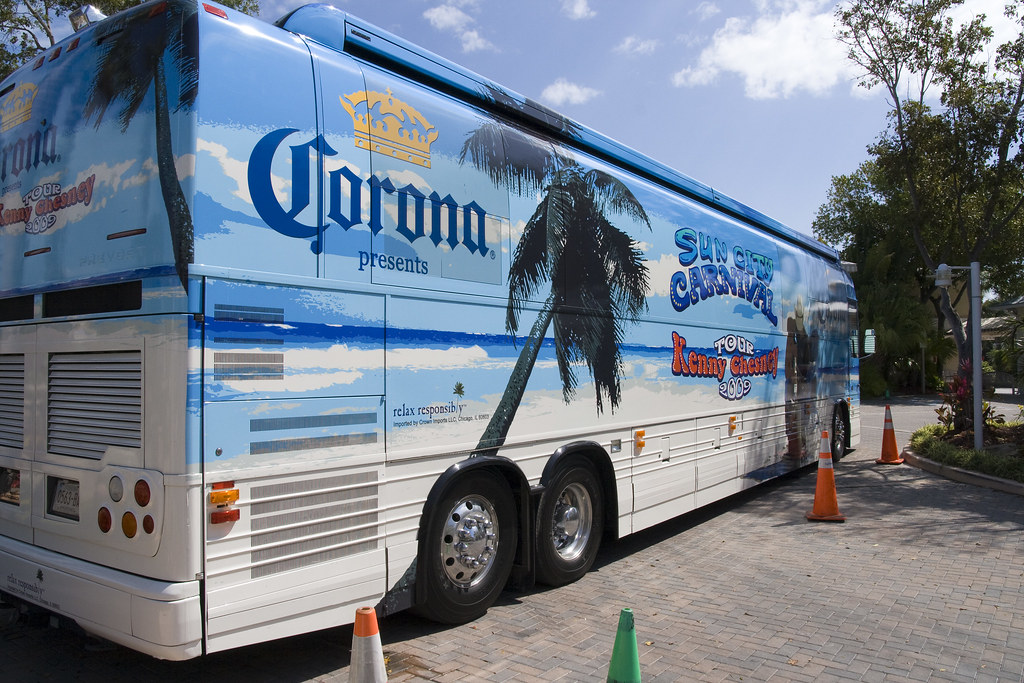A large tour bus, vibrant with a beach-themed mural, is parked in front of a bricked driveway blocked by four traffic cones. The bus, which serves as a concert bus for Kenny Chesney and his band, features a detailed advertisement for the "Sun City Carnival Tour 2009." The upper half of the bus showcases a serene sky-blue background with white clouds, choppy blue ocean waves, and leaning palm trees. The bottom half resembles a sandy beach, tying together the coastal theme. 

Prominent text includes "Corona" with a gold crown logo, the tour name "Sun City Carnival," "Tour 2009," and "Kenny Chesney" in bold red letters. The back of the bus continues this tropical aesthetic, displaying another palm tree with the Corona logo and the words "Relax Responsibly" in black letters. The surroundings include a tree to the right of the bus, grassy areas, a grey light post, and tan structures with brown roofs in the background. The bus is oriented with its front facing to the right, contributing to the lively outdoor and festive atmosphere.